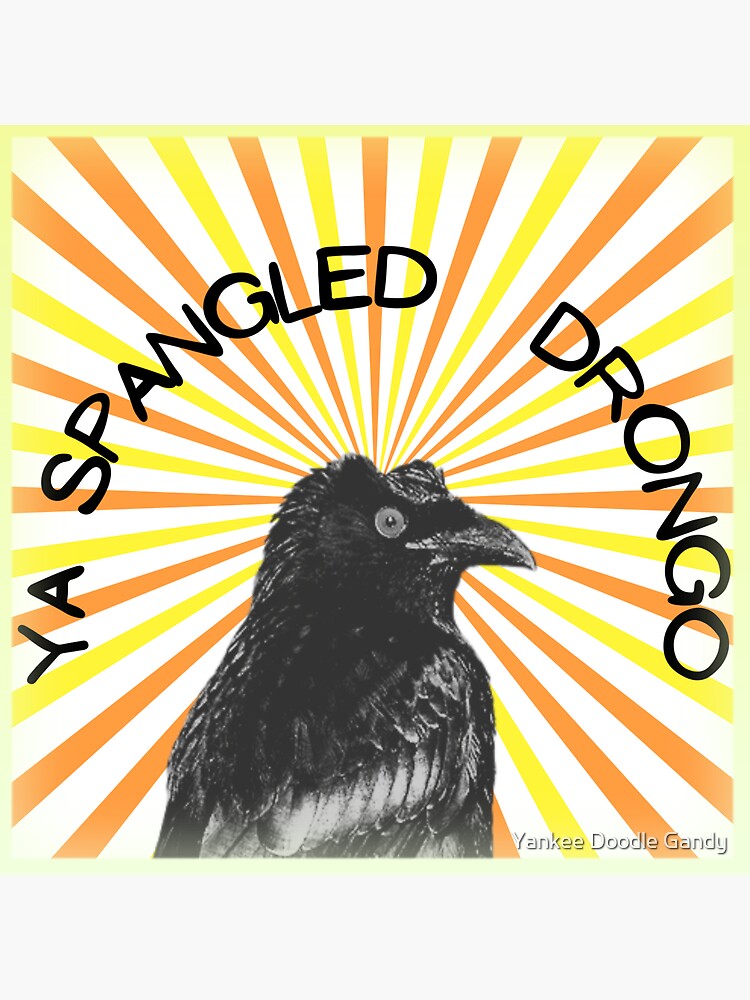This is a square digital illustration depicting a black crow centrally positioned. The crow's head, which is tilted to the right, takes up the center of the image. The eye of the bird is black with a hint of gray, and it has a slightly curved beak. The top of its head appears dented. Radiating from the crow's head are psychedelic lines that create a tunnel effect, reminiscent of 1960s or Brady Bunch imagery. These lines alternate in white, orange, and yellow, and get progressively wider as they move outward from the center. Encircling the crow’s head is the black text "YA SPANGLED DRONGO" in a handwritten style. In the lower right corner, white text reads "Yankee Doodle Sandy." The entire image has a light greenish-yellow border, giving it a contemporary design feel.